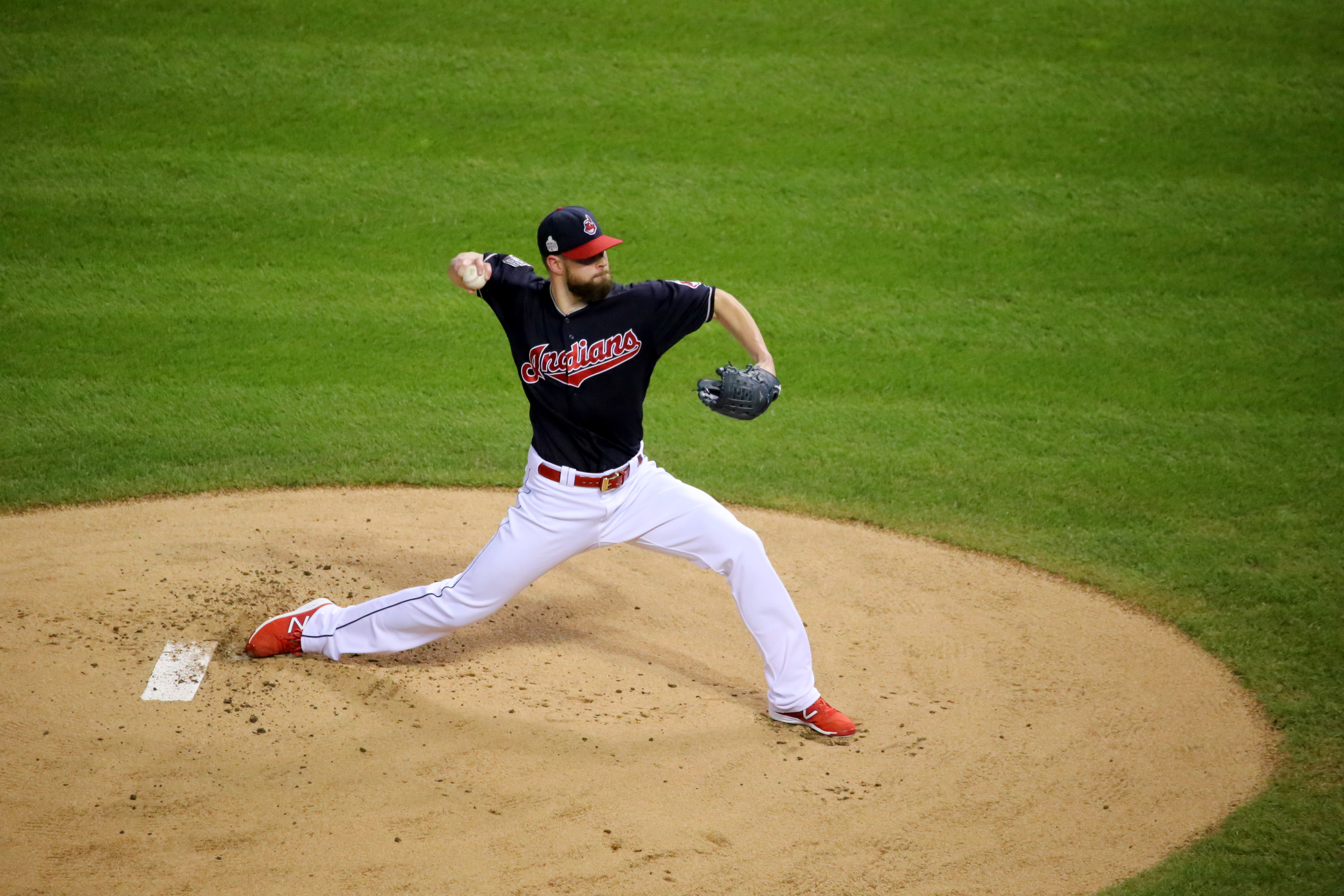This image captures a professional male Caucasian baseball pitcher, mid-motion in the act of pitching a baseball. The pitcher, representing the Indiana Indians, is fully decked out in a navy blue jersey emblazoned with red text reading "Indians," paired with white pants accented by a black pinstripe down the sides. He sports a navy blue hat detailed with red sections and a distinctive Indian emblem, a black glove, a brown belt, and striking red New Balance cleats with a white "N" insignia. Positioned on the pitcher's mound – a circular stretch of tan dirt and sand marked by a white pitching plate – his stance is dynamic; his right leg is extended far behind him while his entire weight is thrusting forward on his left leg. His right arm is cocked back, ready to release the ball, while his left hand bearing the glove is extended in front of him, perfectly capturing the intensity of the moment. The well-maintained field surrounding the mound is lush and green, sporting carefully manicured striped grass. The photograph, likely taken at night, emphasizes both the athlete's focused vigor and the beautifully maintained baseball field.